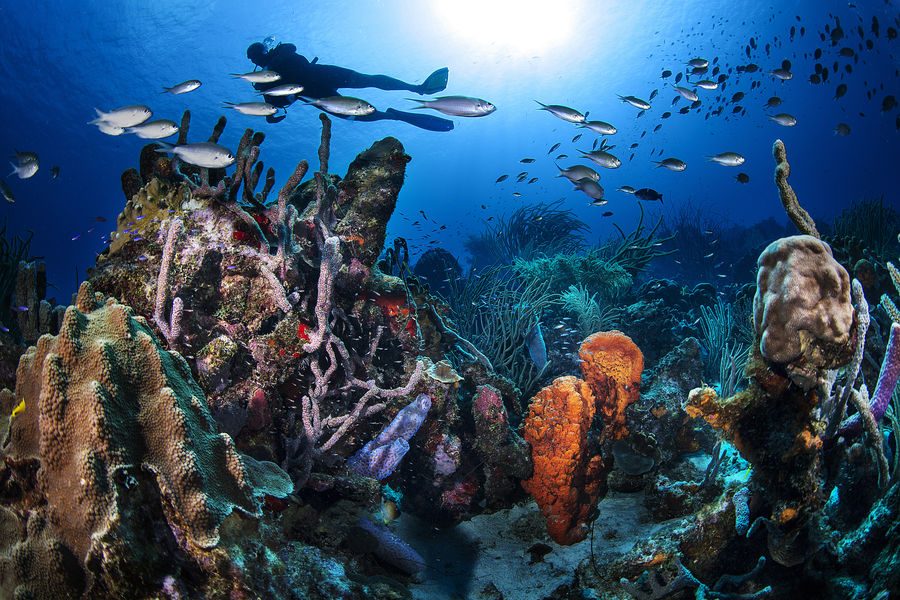An underwater photograph captures a scuba diver in a vibrant coral reef, framed in a rectangular shape with the top and bottom sides twice as long as the left and right sides. The entire scene is submerged under blue-tinted water, giving a serene bluish filter to the photograph. At the top center of the frame, just below the water's surface, an orange sun shines through, illuminating the upper section where a diver in a black diving suit, large fins, and a breathing apparatus can be seen swimming.

The diver appears as a distinctive silhouette, with schools of silver, disc-shaped, and teardrop-shaped fish gliding nearby. Below the diver, the coral reef unfolds into a stunning underwater landscape. On the lower left, a mountain of brown coral, tinged with green at the edges, rises prominently, accompanied by white and blue corals. To the right, a tower-like structure of similarly varied coral stands tall. A striking purple tube-shaped coral stretches from the lower right to the right center, adding vivid color to the scene, while an orange coral branch reaches upwards from the center towards the surface.

Throughout the background, seaweeds sway with the water's currents, adding a dynamic flow to the composition. The reef bustles with marine life, as fish swim both in schools and individually, enhancing the snapshot of this thriving underwater ecosystem. The diver's distant, yet clear presence under the sun's glow ties together this captivating exploration of the wonders beneath the waves.